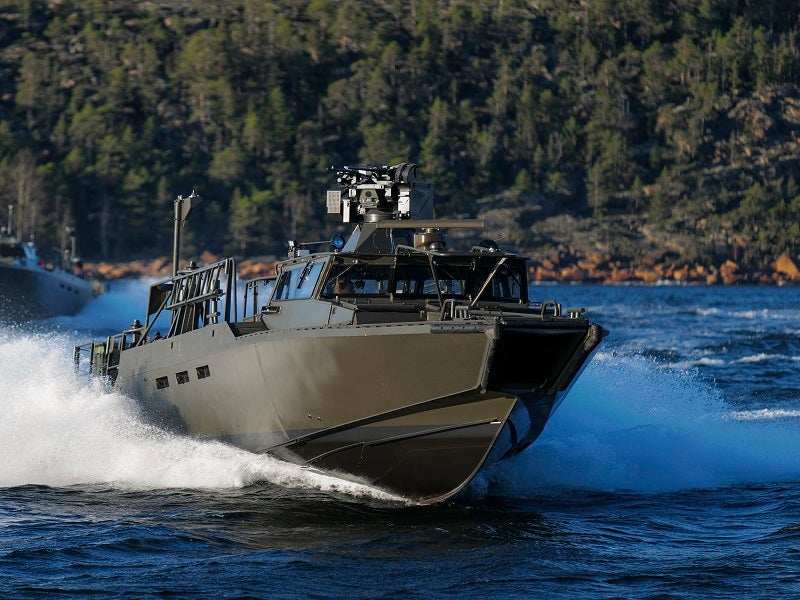The horizontal photograph captures a small, metallic greenish-gray military-looking vessel speeding through vibrant blue, choppy waters. The boat features a small front cabin with thick glass windows equipped with black windshield wipers and appears to be big enough to hold about four people. Its open back is flanked by green railings, and the vessel is fitted with multiple antennas and possibly flashing lights at the rear. Mounted on the roof of the cabin is a large, heavy machine gun accompanied by storage boxes. In the background, a steep cliff face with red buildings suggests the boat is near a small town. Additional details include brownish cliffs and a lush green forest lining the shore, with another vessel visible to the left. The boat is creating a significant wake, adding to the dynamic scene.